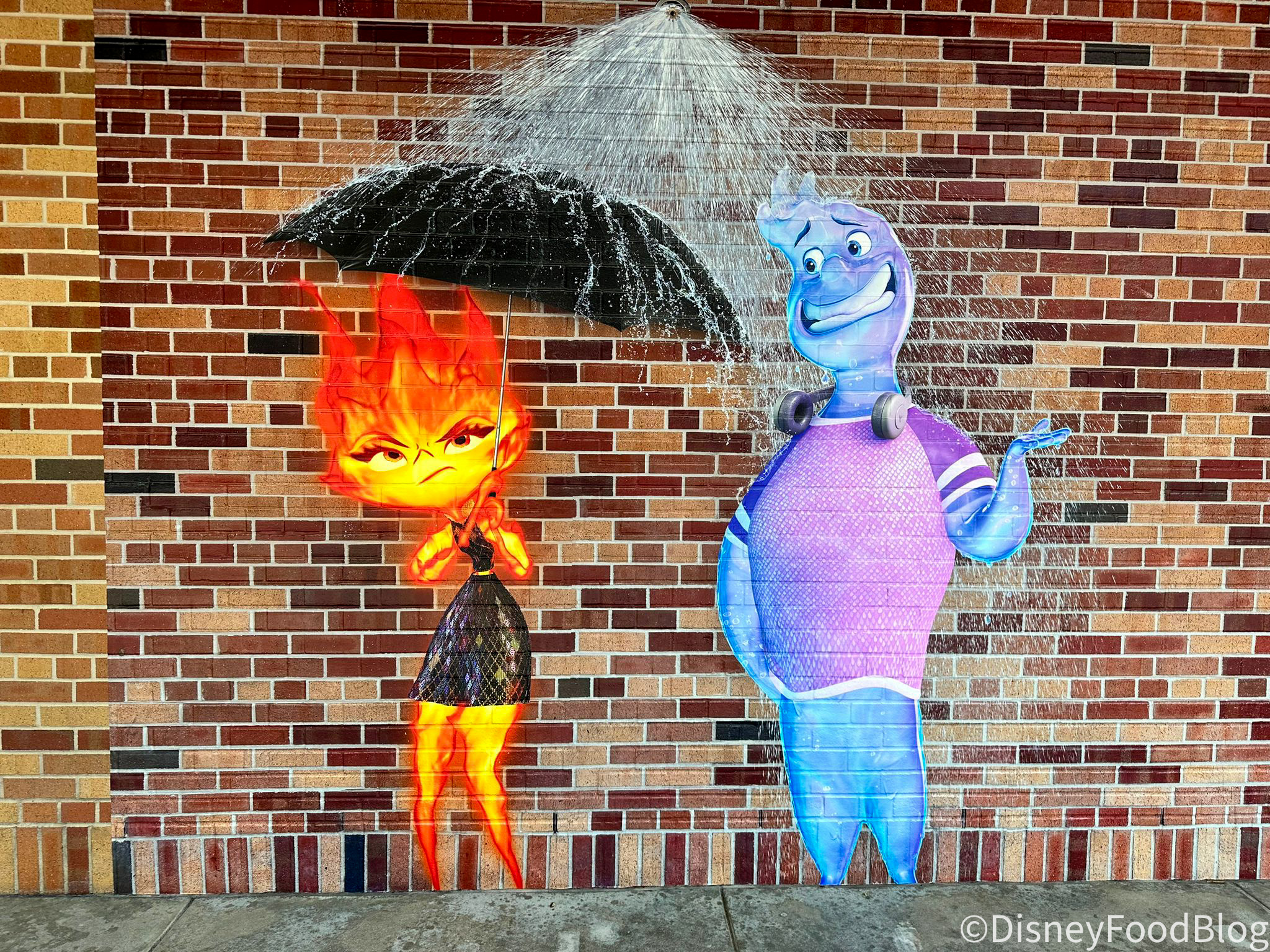This image depicts a vibrant mural on a varied brown brick wall, showcasing two whimsically cartoonish characters personifying fire and ice. On the left, a disgruntled female figure with flames for hair and a yellow face, scrunching her nose in annoyance. Her fiery appearance is accentuated by a spiky red flame head and legs made of fire, complemented by a black sequined mini dress and black high-heeled shoes. She holds up an umbrella to shield herself from the water raining down from a sprinkler above.

To her right stands a cheerful male figure symbolizing ice, exuding a glistening, rounded, and bubbly demeanor. He wears a lavender t-shirt adorned with white stripes on the sleeves and sports headphones around his neck. With a big smile on his face, he lifts his left hand in a friendly gesture towards the fire woman, seemingly enjoying the water showering over them from the sprinkler above. The mural creatively contrasts their elements, capturing a humorous and dynamic interaction between the playful ice man and the fiery, disgruntled woman.